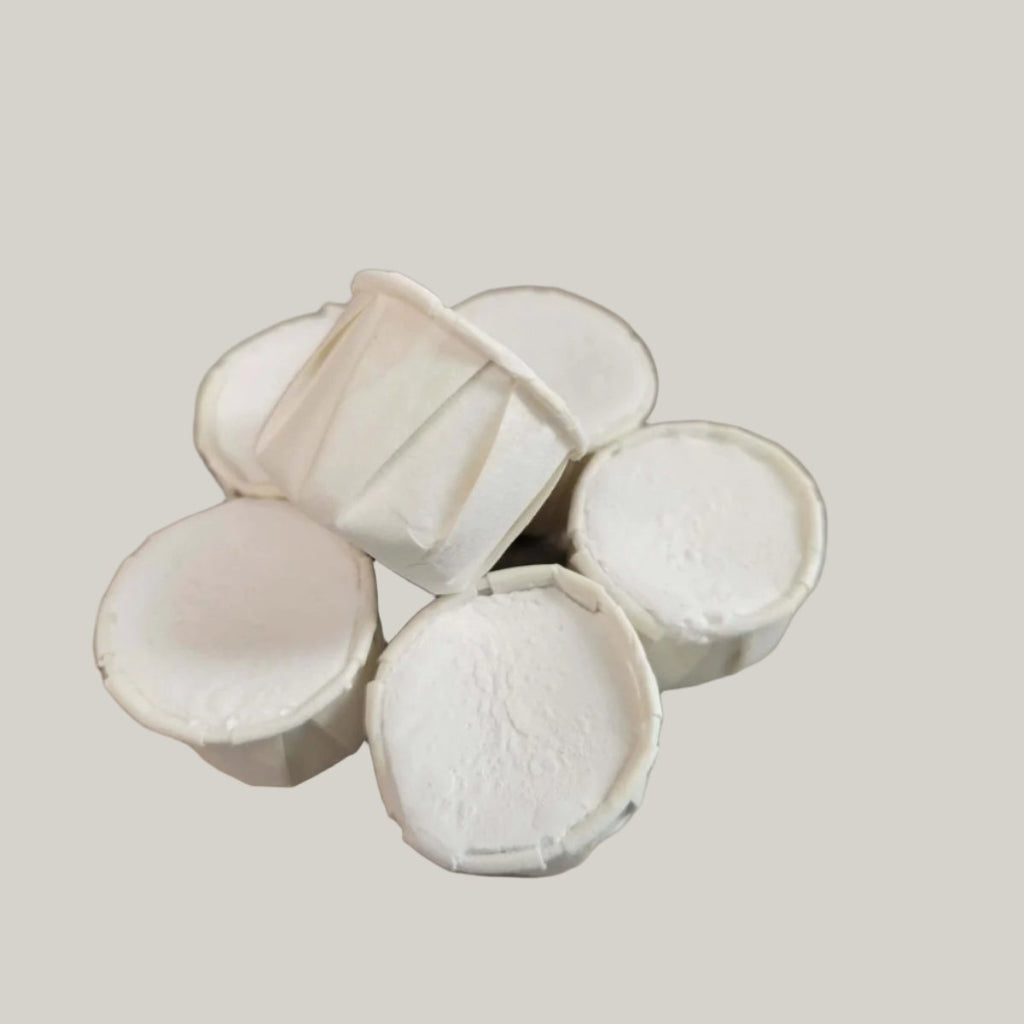The image features six small white paper condiment cups, typically found in restaurants for serving sauces or condiments. Five of these cups are arranged in a circular pattern on a gray, cracked concrete surface, resembling a flower shape. One additional cup lies tilted on its side atop the circular arrangement. Each cup is filled with a smooth, thick white substance that could be sour cream, cream cheese, or a similar paste. In the background, there is a green bowl with legs, often seen in Mexican restaurants for serving salsa, along with a brown splotch and a cluster of yellowish-brown triangular objects. The setting appears to be an outdoor seating area at a restaurant.